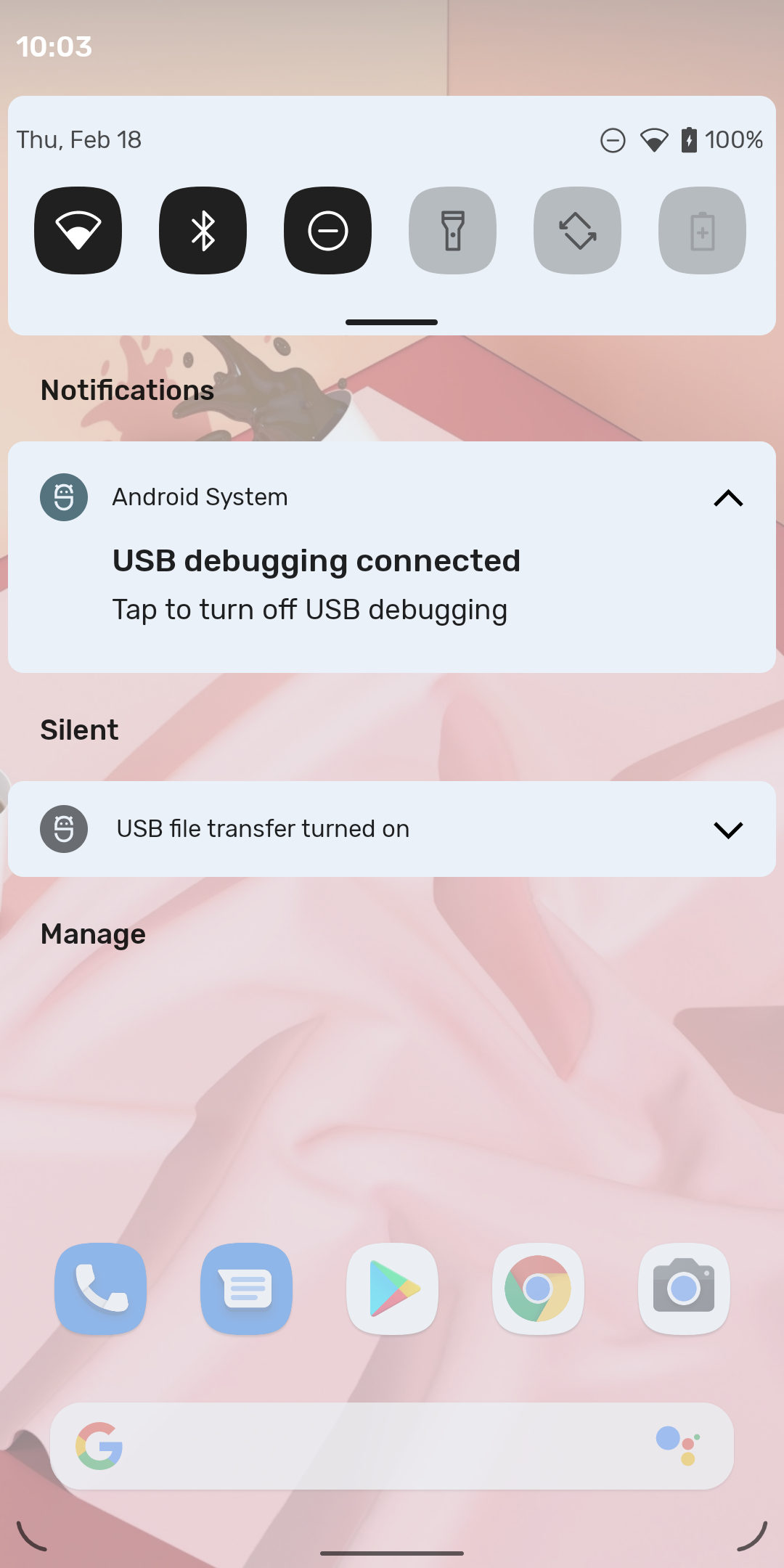This is a detailed screenshot of an Android home screen with the notification shade pulled down, revealing various details. At the top left corner, the time is 10:03, displayed in white text. Below the time, in a gray rectangular box, the date is shown as Thursday, February 18th. The phone is currently charging at 100%, indicated at the top right. The device is connected to the internet and set to "Do Not Disturb" mode, denoted by the corresponding icons.

Below the date and charging information, there are six toggles: the left three show active connections to the internet, Bluetooth, and "Do Not Disturb" mode, while the right three show the flashlight is off, auto brightness is enabled, and battery optimization is not active.

Underneath these quick settings, there are notifications. One notification from the Android system indicates that USB debugging is connected, with an option to tap and turn off USB debugging. In the silent notifications section, it mentions that USB file transfer is turned on. There's also an unclickable "Manage" option.

The phone's background features a piece of basic artwork. At the top, a cup of coffee appears to be spilling, and below it, there's pinkish fabric with hints of red. The home screen also includes various apps and a Google search bar.